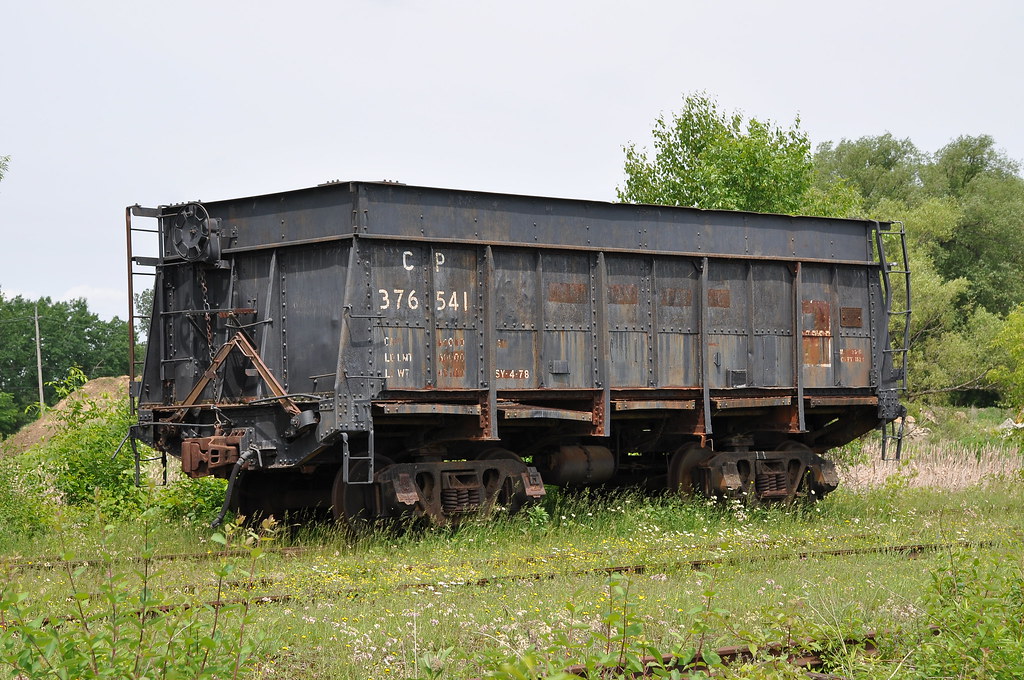The image showcases an abandoned rusted train car that bears the faded white text "CP-376541." This horizontally aligned rectangular photograph captures the train car centered in the middle, with its dark gray and streaked brown surface signifying its age and neglect. Below the car, old overgrown train tracks and tall grass, dotted with small white flowers and dandelions, stretch across the foreground. The right side of the background is dominated by tall trees, while the left side features more distant trees and a power line. Overhead, a light gray, cloudy sky forms the backdrop, enhancing the desolate atmosphere of the scene.